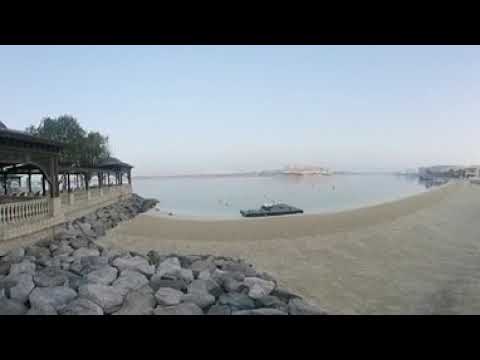This is a detailed photograph capturing a serene shoreline scene. In the center of the image, on the calm water, there is a small black watercraft near the shoreline. The shoreline is bordered by light tan sand leading up to a cluster of rough gray rocks on the left. Among these rocks, there is an elegantly designed structure resembling a covered platform or gazebo, which might serve as an outdoor restaurant. This structure features a dark wood roof supported by wooden columns and is partially enclosed by gray stone barriers. Surrounding the platform are lush green trees. In the distance, on the right side of the image, there are housing units that appear white and gray. The expansive sky is predominantly white with patches of blue on either side, framing the tranquil waters and sandy beach below. The overall scene is peaceful and picturesque, likely capturing an outdoor beach setting with potential hospitality amenities.